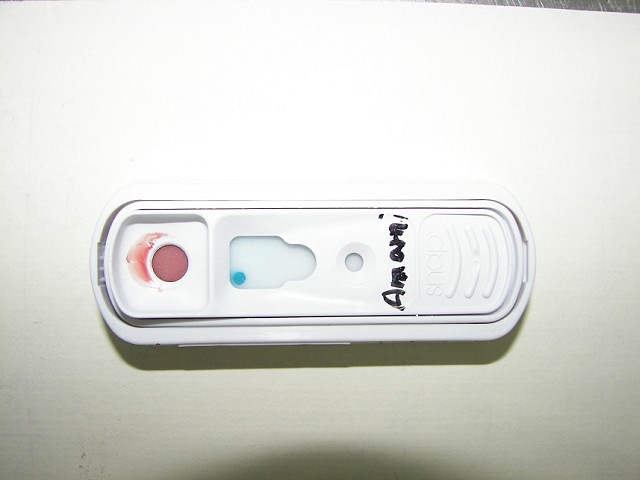This horizontal image showcases a plastic testing device on a white sheet of paper. The device is segmented into three distinct sections and features a raised, thick structure. Positioned at the top left (considering the device is turned perpendicular to the viewer's perspective), there is a circular area marked by a purplish-red color. Adjacent to this is a bridge-shaped indentation leading to a smaller rectangular section, which contains a blue dot located at its lower left corner. To the right of this section lies a smaller circular opening, intended for placing a sample. The device includes a semicircular arc with finger grips at the far right end of the test area, facilitating handling. Handwritten in black Sharpie below the small circle where the sample is applied is the word "amen."